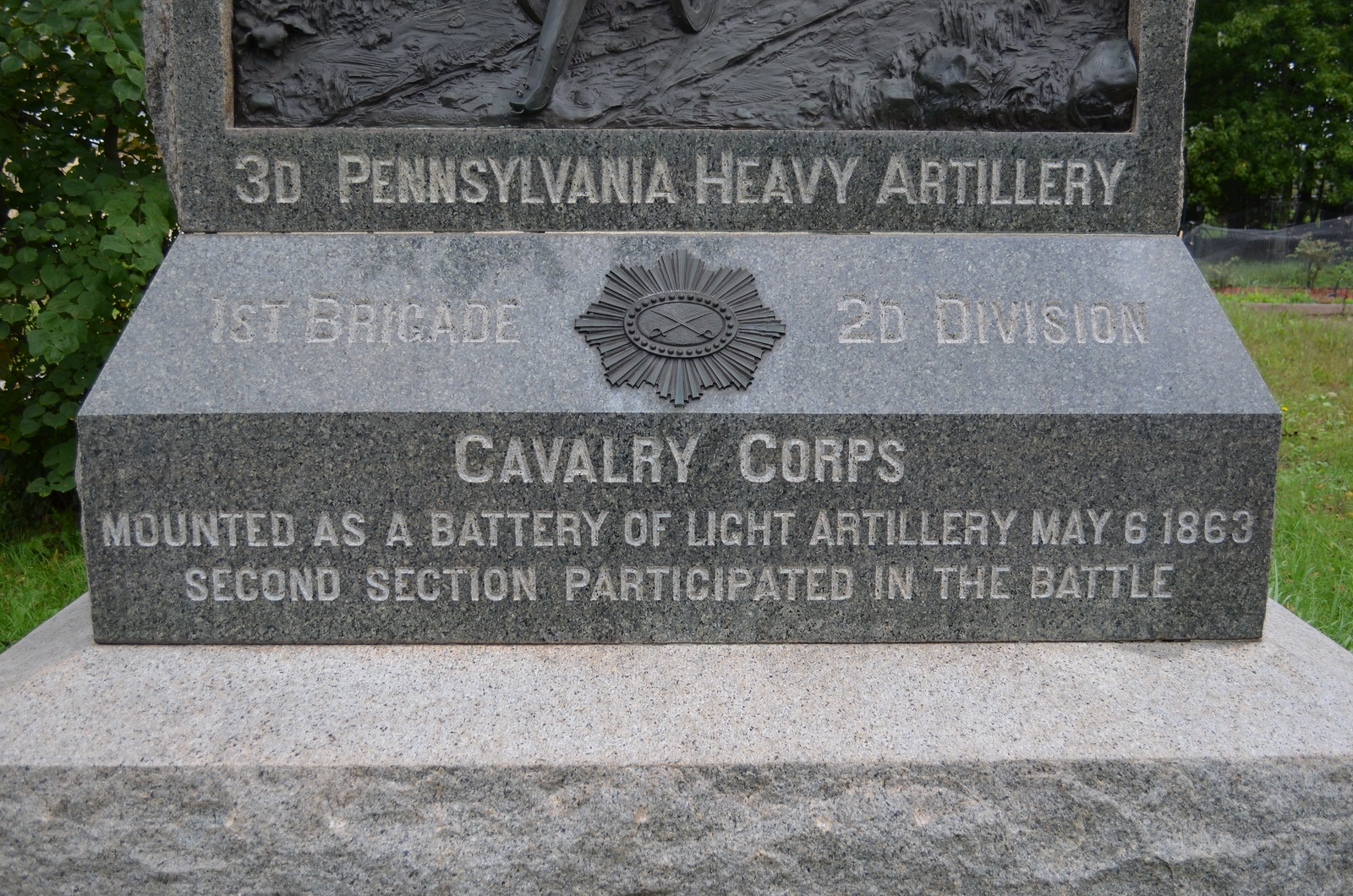This image showcases a close-up of a granite historical marker set in an outdoor park area, distinguished by a manicured lawn and trees in the background with subtle sunlight filtering through, indicating it was taken during the daytime. The monument itself is predominantly gray and features intricate chiseling. At the top, there is a bronze inset panel, partially visible, with the engraving "3D Pennsylvania Heavy Artillery." Below this, on the flat panel, it reads "1st Brigade," followed by a metal emblem and the inscription "2D Division." Further down, it states "Cavalry Corps, mounted as a Battery of Light Artillery, May 6, 1863, second section participated in the battle." This entire structure sits on a beveled, lighter-colored granite base, providing a stable and prominent foundation. The encompassing area of the park with its greenery suggests a calm and respectful setting appropriate for reflection on historical events.